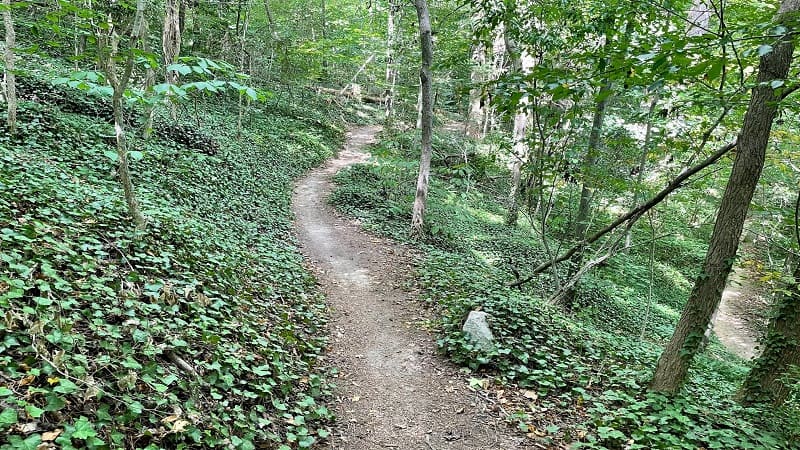This is a detailed photograph of a narrow dirt path winding through a dense forest, rich with natural beauty and intricate details. The path, designed for nature walks or hikes, splits the image as it meanders deeper into the woods, flanked by a variety of trees with thin barks and a wealth of green foliage. On either side of the trail, the ground is covered with low-hanging leafy plants, short greenery, ivy, and some small weeds, creating a lush, green groundcover that is both vibrant and abundant. Scattered along the path and within the surrounding greenery are natural elements such as sticks and a rock, adding to the rugged, untouched feel of the area. One tree has fallen over, emphasizing the natural, unmanicured environment. Sunlight trickles through the canopy, casting light and shadows on the path below and enhancing the tranquil, serene atmosphere of this secluded natural setting. In the right-hand corner of the image, another part of a trail can be seen, suggesting a network of paths within this forested area. The photograph captures the essence of a quiet, solitary trail inviting further exploration.